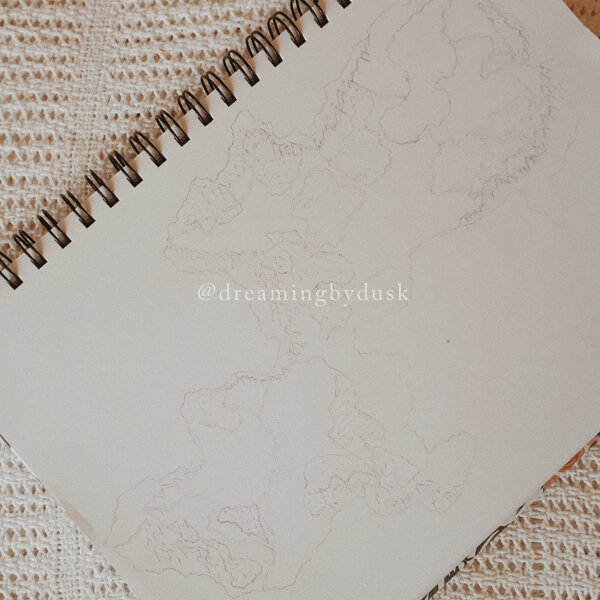The image features a spiral-bound sketchbook diagonally positioned atop a white or off-white crocheted blanket, reminiscent of a doily. The sketchbook's black double-spiral binding casts distinct shadows upward and to the left. Within the sketchbook, a faint pencil drawing depicts what appears to be a topographical map, showcasing two interconnected landmasses—one larger in the top corner and a smaller one in the bottom left. The scene is muted with predominantly white and off-white tones, contributing to a faded, delicate atmosphere. Central to the image is a watermark reading “@ Dreaming by Dusk” in white text.